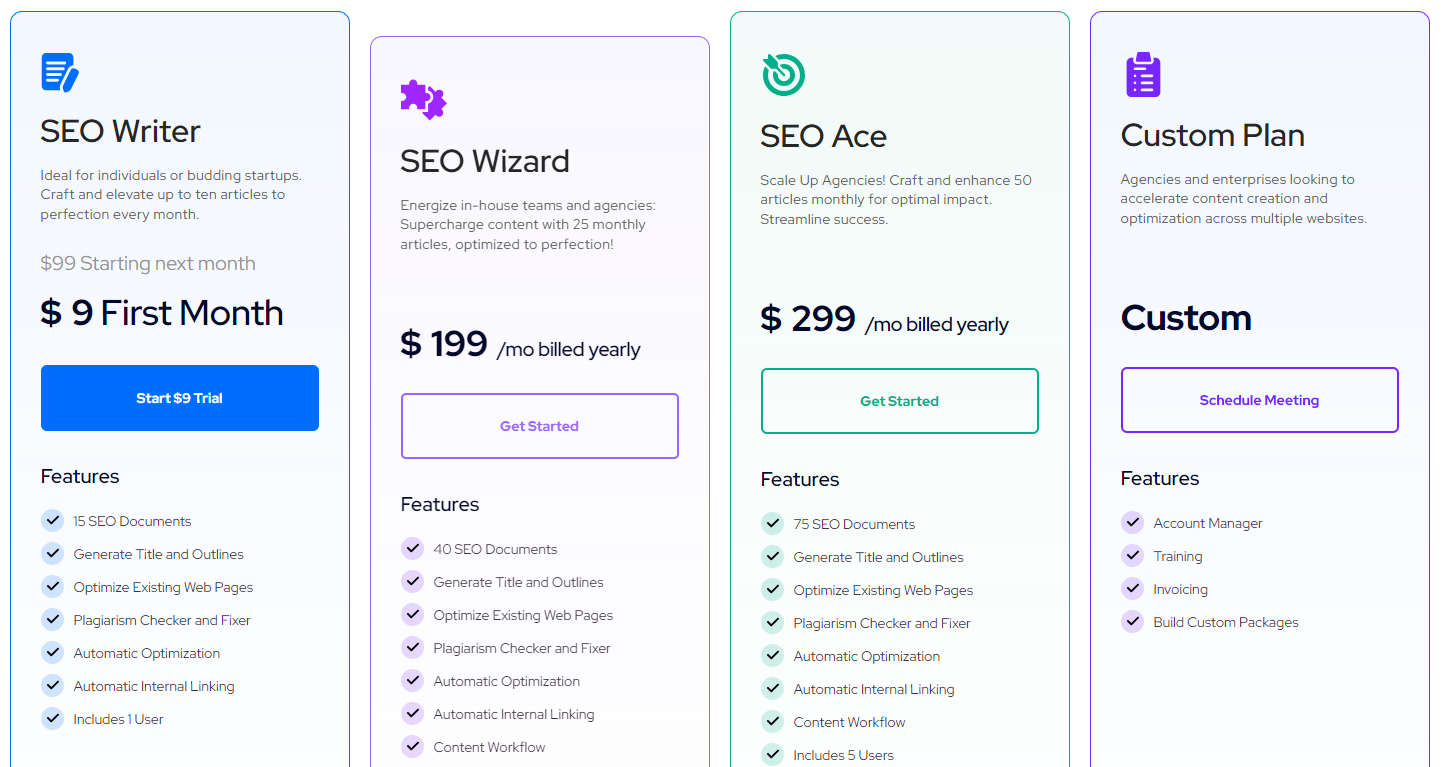The image is divided into four areas, each comprising a central button, a top section, and a feature section at the bottom. The leftmost area has a light blue background and displays an icon of a piece of paper and pencil at the top. Below the icon, it reads "SEO Writer," described as ideal for individuals or budding startups. The service promises to help craft and elevate up to 10 articles to perfection every month, priced at $99 monthly, with a promotional rate of $9 for the first month. Under this description is a dark blue button labeled "Start $9 Trial." Below the button, in a smaller, somewhat blurry font, it lists additional features: "Feature 15 Documents," "Optimize Existing Webpages," "Plagiarism Checker and Fixer," "Automatic Optimization," and "Automatic Internal Linking."